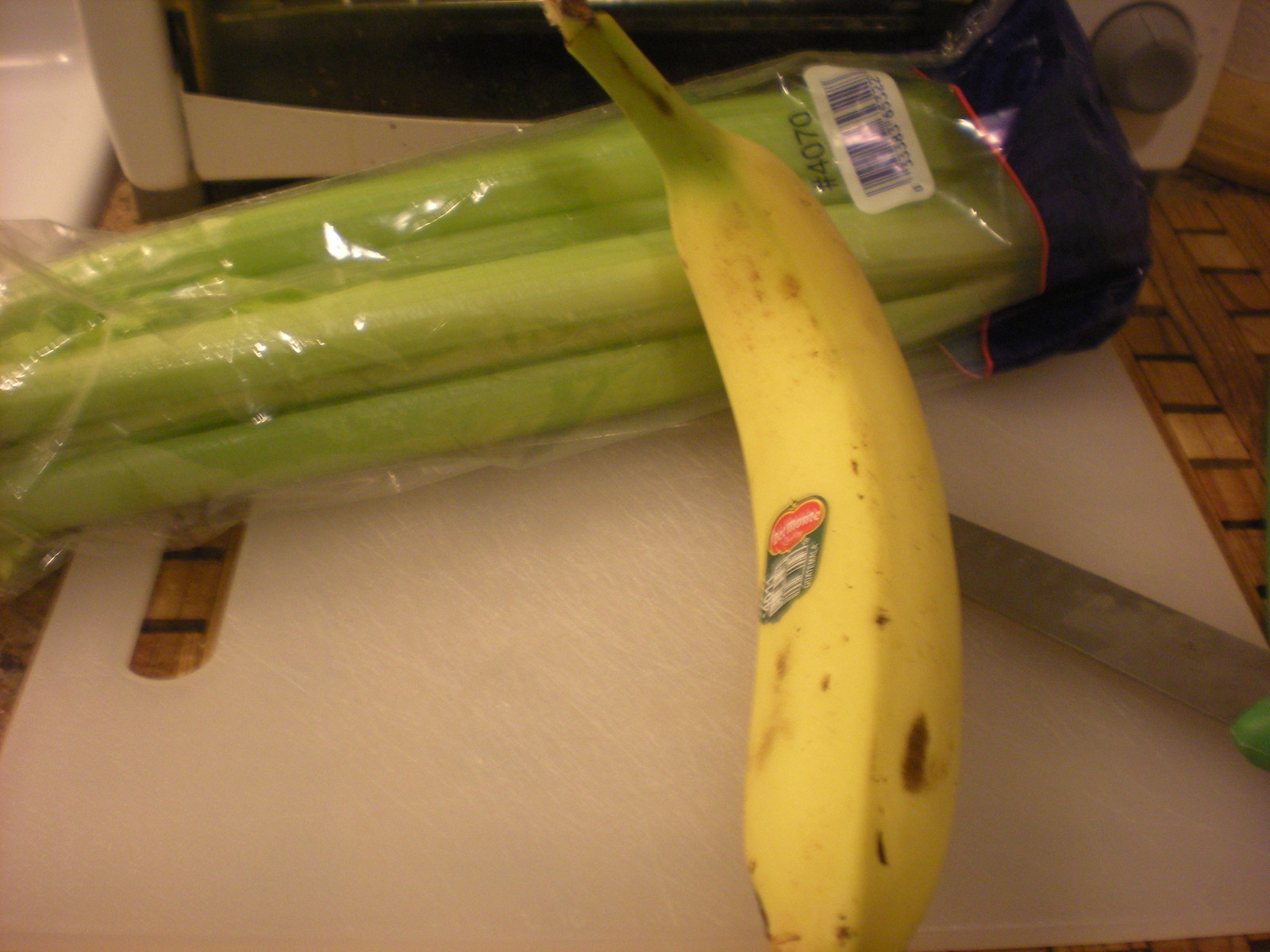The image captures a detailed scene on a kitchen countertop featuring a fresh banana and a bag of celery. The banana is positioned vertically, leaning slightly against the celery, which remains inside its bag and laid out horizontally across a white plastic cutting board. The cutting board itself is positioned horizontally on a countertop composed of small mosaic tiles. Notably, the banana sports a Chiquita label and has a small brown spot on its right side, indicating it is at its peak ripeness. A knife appears to be nestled underneath the banana. In the background, the upper portion of a microwave or toaster oven is visible, cropped at the very top edge of the image.